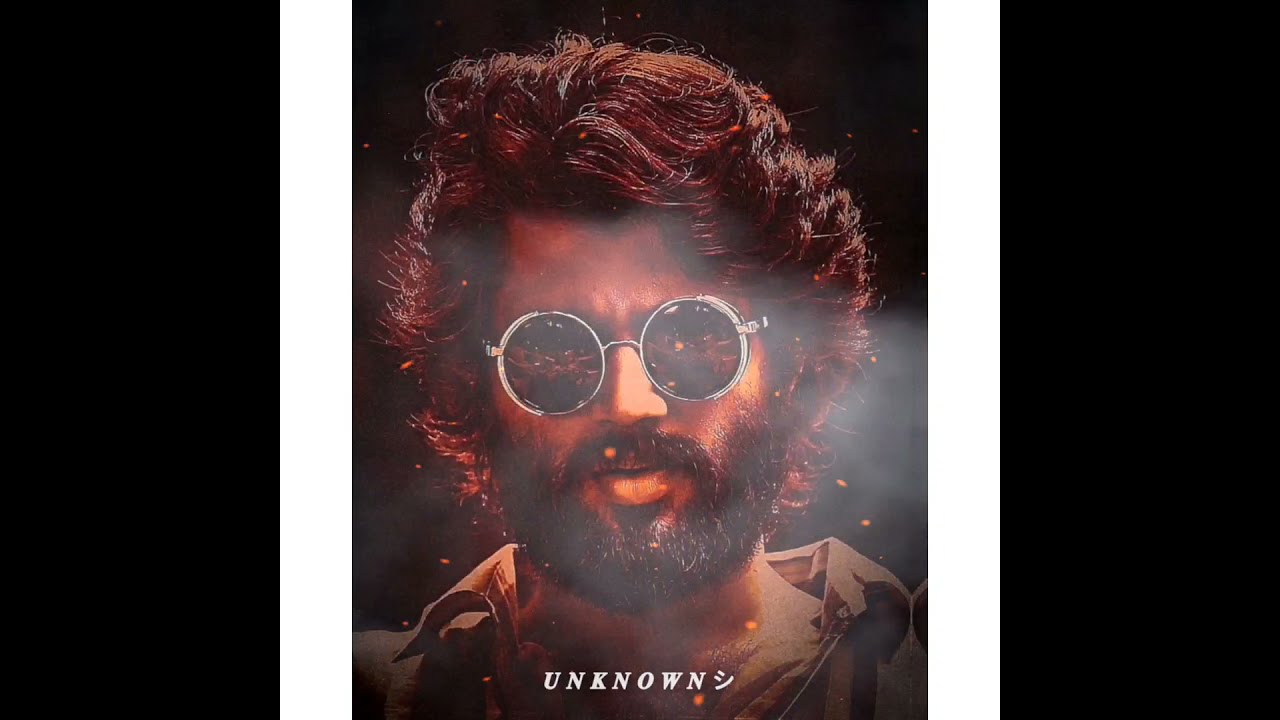The image is a highly stylized, animated portrait that could easily be the cover of an album. It is divided into three main sections: a black rectangular box on the left, a black rectangular box on the right, and a central area featuring the portrait of a man. The left and right black sections are separated from the central portrait by thin white vertical lines. The man, who appears to be of Indian or Pakistani descent, has dark brown, wavy hair with hints of red and a thick, full beard and mustache. He is wearing round, metal-framed sunglasses with highly reflective lenses that have a hint of red, and a brown button-down shirt. The background of the central section is black, overlaid with a smoky fog and scattered orange embers, adding to the overall dramatic effect. At the bottom of the portrait, the word "unknown" is displayed in white text, accompanied by a Japanese symbol.